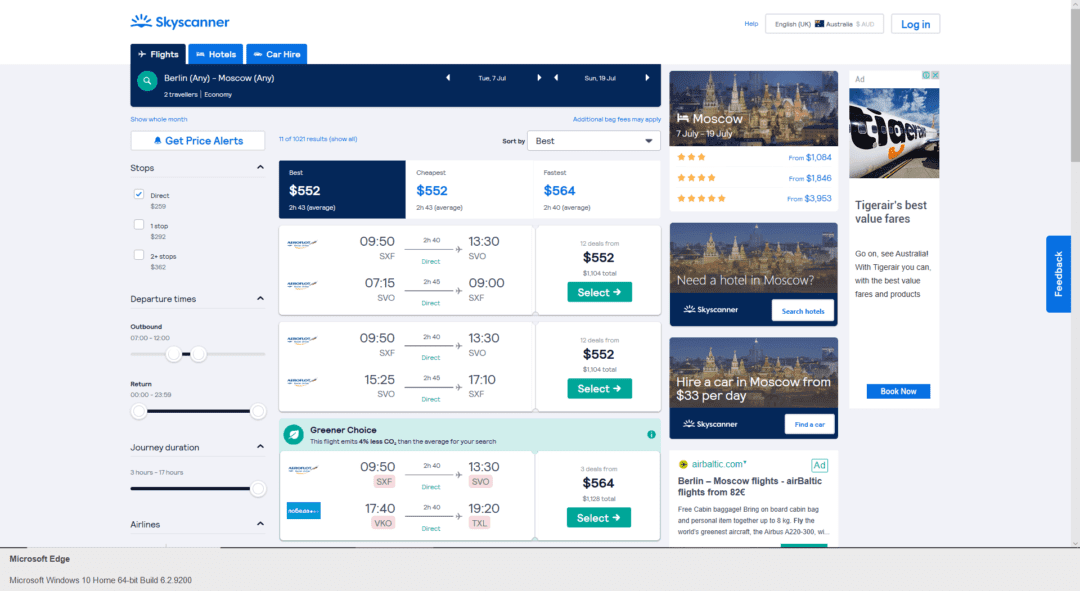This image is a screenshot from the Skyscanner website. The website's header is primarily blue, featuring a logo that resembles a blue sun. Below the header, navigation tabs labeled "Flights," "Hotels," and "Car Hire" are displayed. 

Beneath these tabs, a black bar stretches across the page, containing a white box that prompts users to "Get Price Alerts." Below this bar, there are several blue price boxes indicating flight costs, such as $552 and $564. This section also includes departure and arrival times for various flights, along with a note on "Greener Choice" for more sustainable travel options.

Each price box has a green "Select" button underneath it, allowing users to choose their preferred flight. On the right side of the image, there are pictures of Moscow's iconic architecture, which resemble ornate castles. Accompanying the images, there are promotional texts such as, "Need a hotel in Moscow?" and "Hire a car in Moscow from $33 per day."

Additionally, there is a section labeled "Tagere's Best Value Fares," featuring an image of a sleek, fast white train with black lettering. Below this, there's a brief mention of Brazil and a reference to "Moscow flights air battle flights," indicating prices starting with a figure that includes the number two.